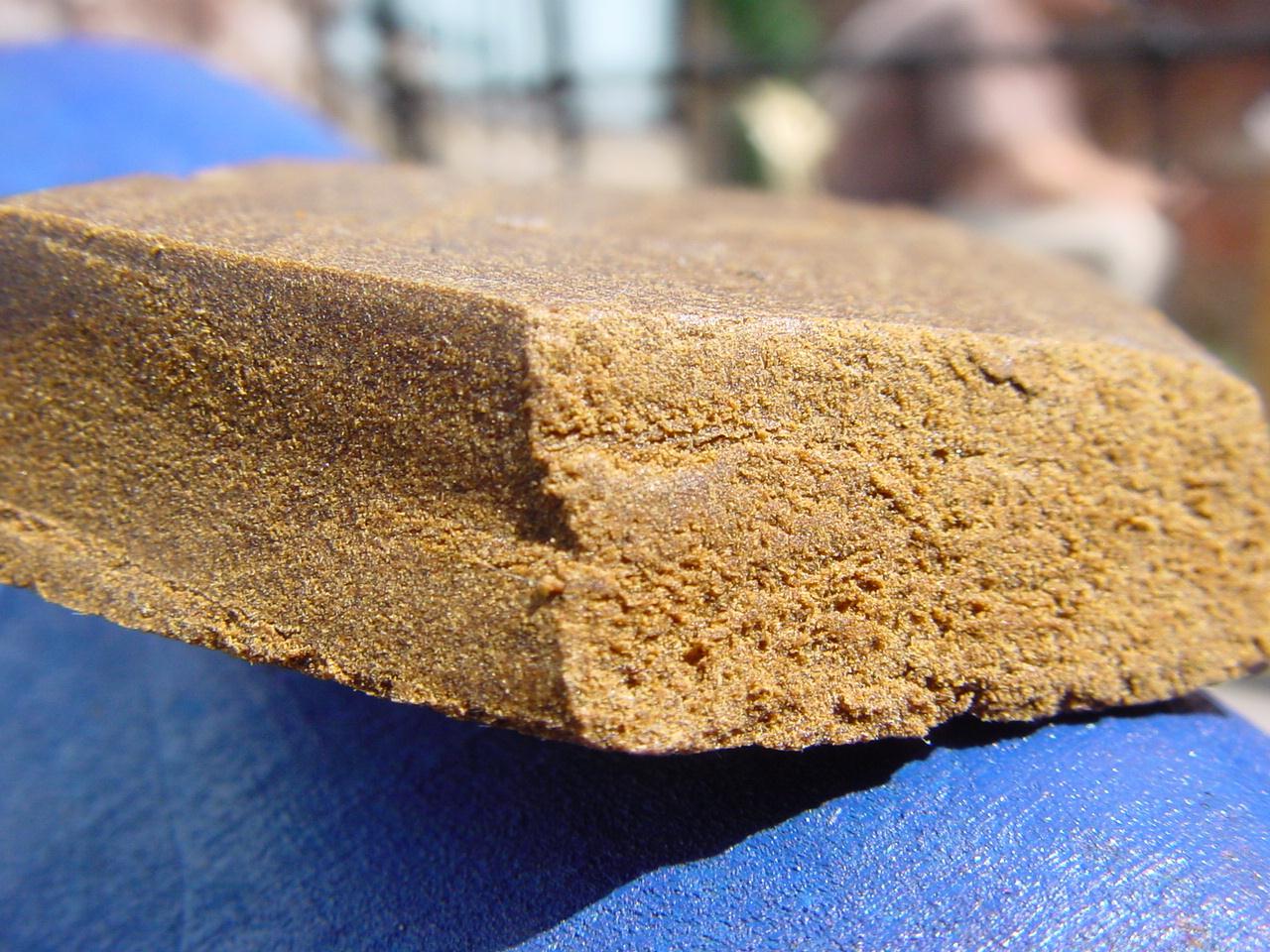The close-up photograph showcases a large, square-edged, golden-brown object with a texture that resembles either hashish, a piece of crumbly pumpkin or ginger bread, or a sand-like candy. This gritty and grainy object has a moist and dense interior with noticeable crumbs along the sides, suggesting it has been cut recently. It rests on what appears to be a painted blue concrete surface. The blurred background gives hints of an outdoor setting, possibly in sunlight, with a touch of green at the top center and a pinkish hue at the top right. There’s also an indication of a sandy-colored ground and a fence, contributing to a beach-like atmosphere.